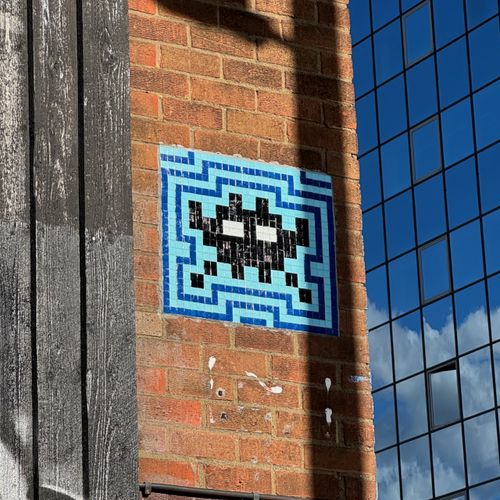This is a detailed color photograph capturing an urban streetscape. Prominently featured is a brick wall adorned with tile graffiti that resembles an 8-bit video game character, reminiscent of Space Invaders. The central figure of the graffiti is a black 'invader' with two distinct white square eyes. Surrounding the black figure is a mosaic of blue tiles, creating a striking contrast against the burnt orange-red bricks of the wall. To the left of the brick wall, three weathered wooden planks, vertically arranged, show signs of age with white speckles and a washed-out appearance. The composition is further enriched by the shadow of a streetlight falling next to the graffiti on the right. Dominating the far right of the photograph is a modern glass building with fully windowed walls, some panels reflecting the clouds in the sky. One of the windows is slightly open, and the squared design of the building's windows cleverly mirrors the pixelated squares of the tile graffiti, creating an intriguing visual harmony.